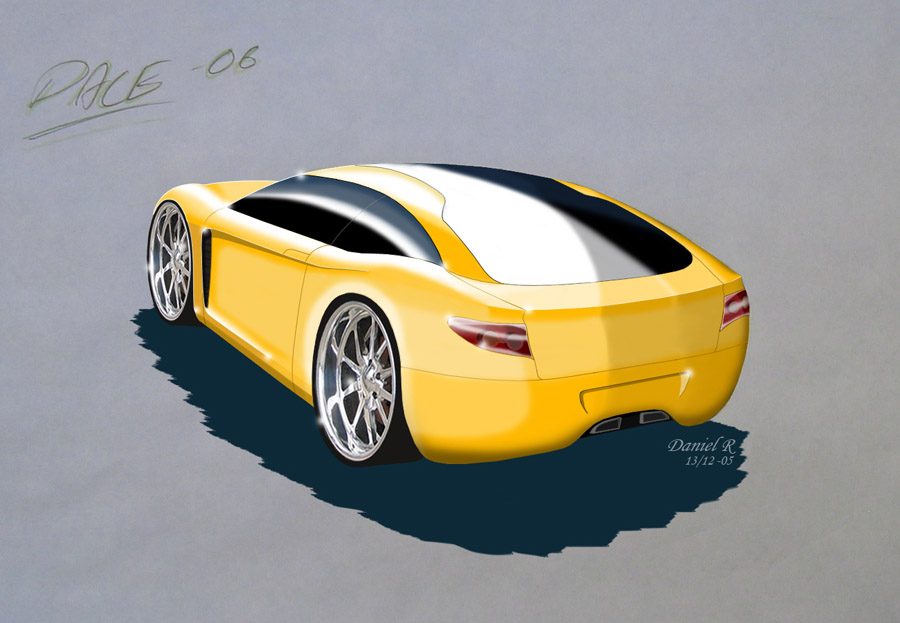This image is a digital print of a sleek, sports car, reminiscent of a Porsche. The two-seater vehicle features two doors and large tires with prominent silver rims. The perspective reveals the side and back of the car, showcasing its aerodynamic and rounded design. 

The car's windows form a continuous, tinted arc from the front windshield, seamlessly sweeping over the top to the rear windshield. The side windows are also tinted and extend from the front to the back. 

The car's taillights are elongated and widely spaced apart. It has a dual exhaust system, yet lacks a visible license plate. 

In the image's background, a shadow effect appears with the text "Daniel R 13/12-05" embedded within it on the left side. Additionally, there is a handwritten note in pencil, which seems to say "DACE 06," and it is underlined.